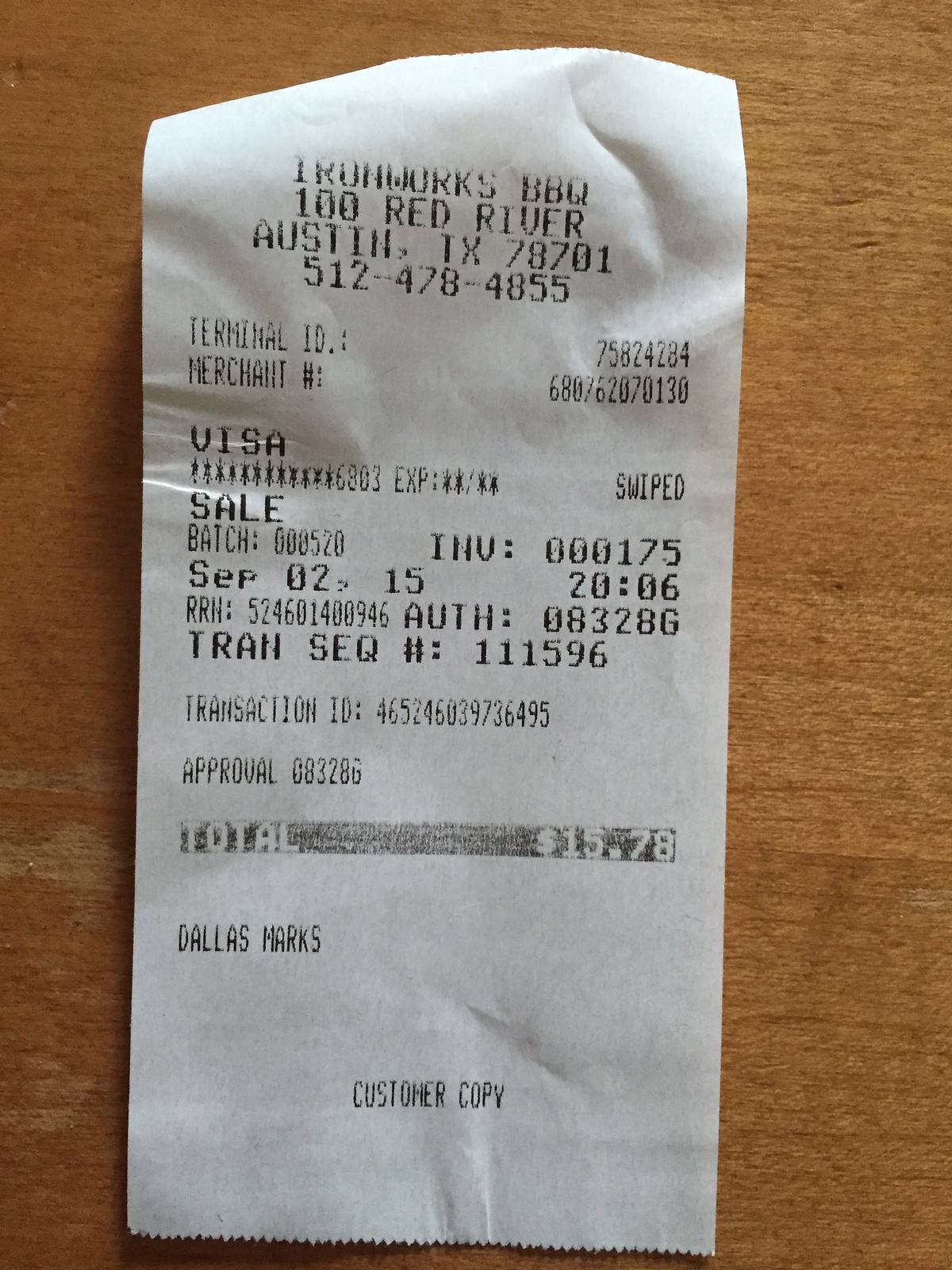A detailed photograph showcases a white receipt from Ironworks BBQ, conveniently placed on a thin, inexpensive wooden table. The receipt, adorned with black text, details a transaction from the establishment located at 100 Red River, Austin, Texas 78701. The contact phone number, 851-247-8485, is also prominently displayed. Essential transaction details are provided, including terminal ID, merchant number, and evident use of a Visa card, indicated by masked digits and expiry details. The card was swiped, leading to a sale recorded in batch number 00520 and invoice 00175. This transaction occurred on September 2, 2015, at 20:06 hours. Additional specifics such as RR number, authorization number, transaction sequence number, and a lengthy 12-digit transaction ID number are documented. An approval number confirms the total amount of $15.78 spent. The receipt bears the name "Dallas Marks" and succinctly denotes "Customer Copy" at the bottom.